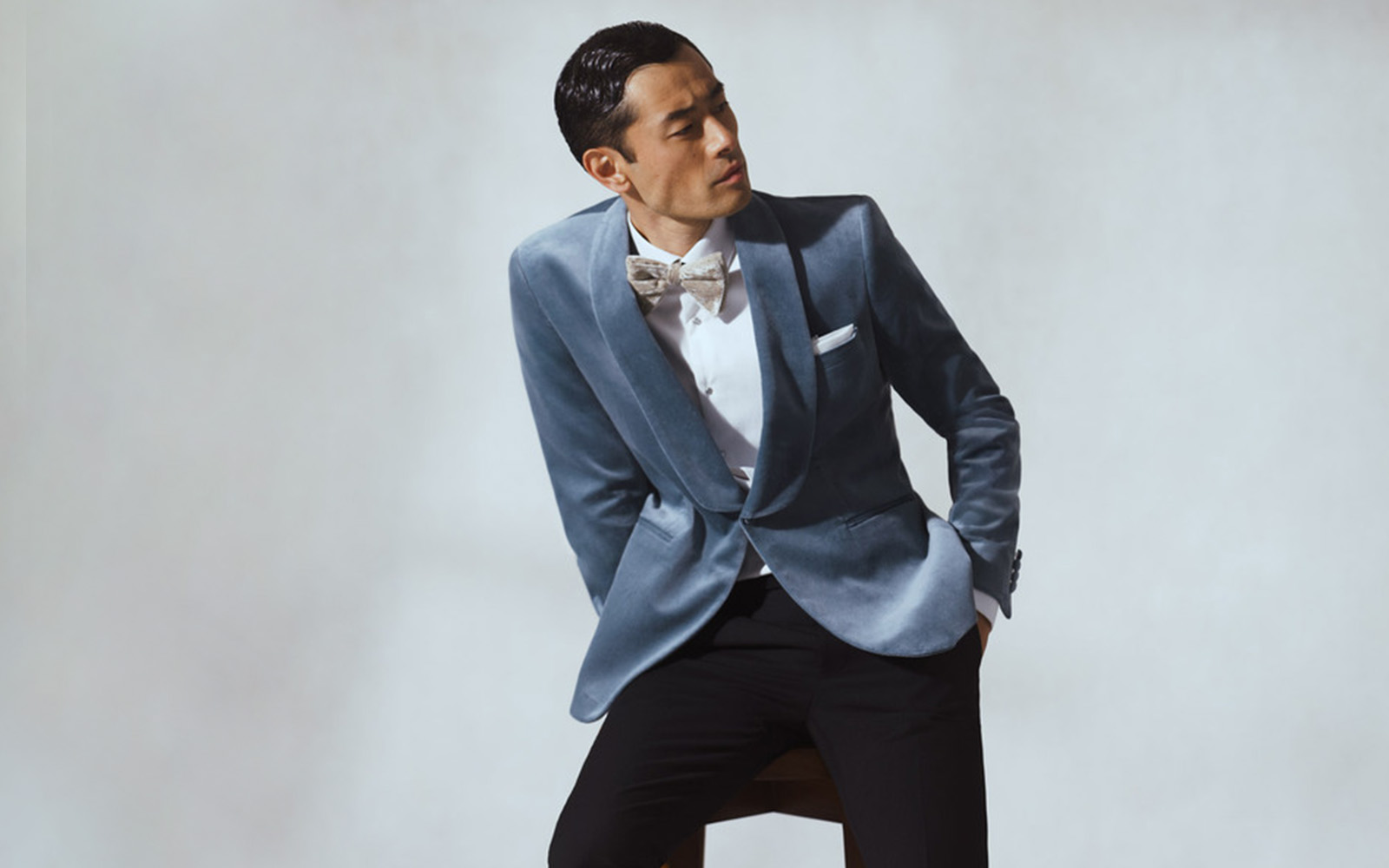In this horizontally aligned rectangular image, we see the front side of a well-dressed man centered against a solid background. The backdrop appears to be a light to medium gray or potentially a blue hue, giving the overall scene a composed, formal tone. The man, who has slightly darker skin and short black hair that looks gelled down, is wearing a sophisticated outfit. His attire includes a suit jacket that might be gray or a satin-like blue—details are unclear—paired with black pants. The jacket is buttoned and features a white collared button-down shirt underneath, accessorized with a light brown or gray-colored bowtie, adding a stylish touch. 

A white handkerchief peeks from his coat pocket on the chest, accentuating his polished look. He is posed with his hands in his pant pockets, and although his full legs are not visible, it seems he might be in a sitting position, possibly on a stool. The man has a thin, sculpted face with a serious expression, and his head is turned towards his right, making his eyes less distinguishable, almost as if they are closed. This detailed portrayal captures a formal and somewhat pensive mood, emphasizing the elegance and refinement of the man's appearance.